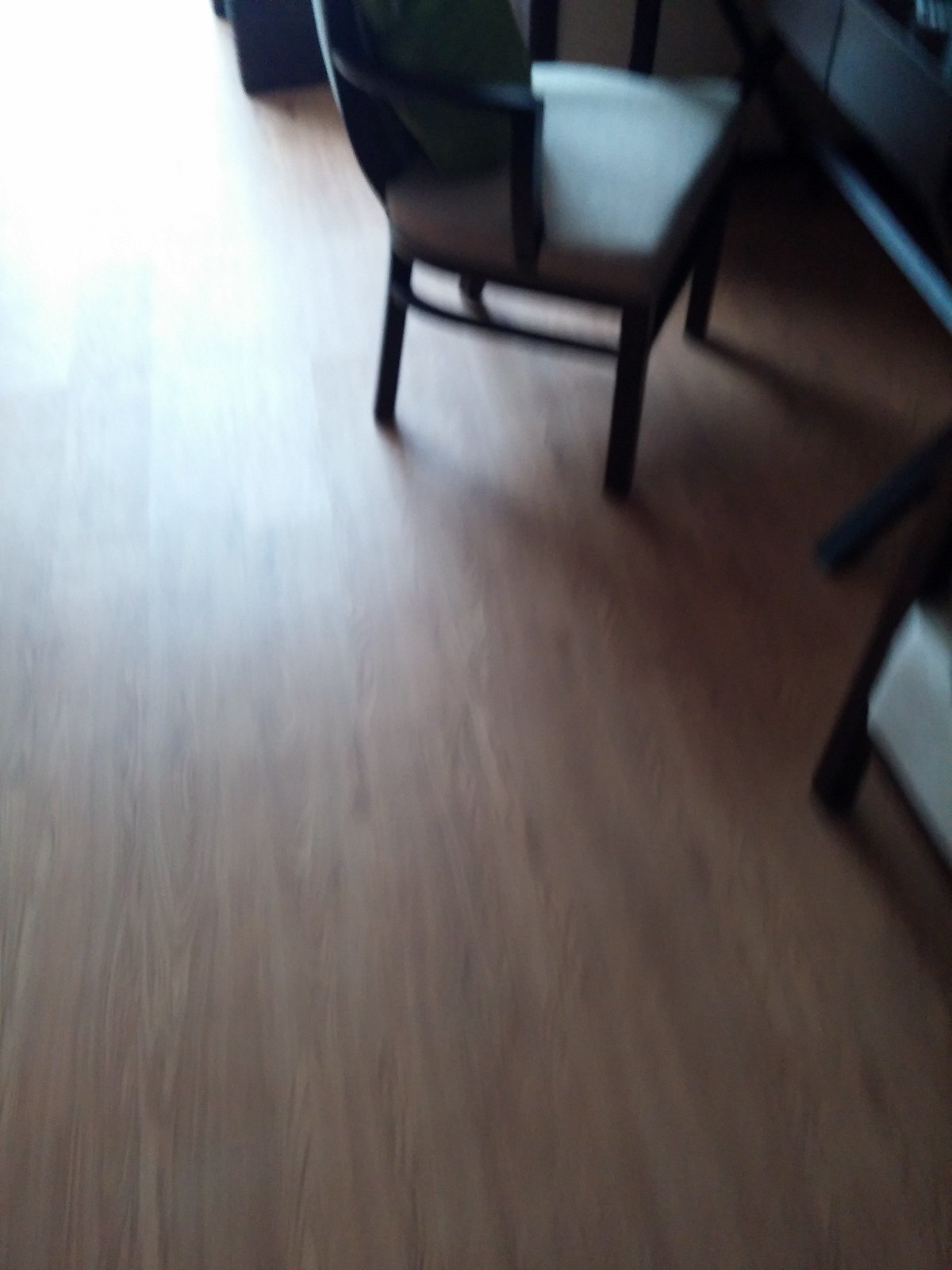In this somewhat blurry and dimly lit photograph, a polished hardwood floor indicative of a professional setting stretches across the space. Centered in the photo is a sleek, black wooden chair adorned with a gray cushion and backrest, positioned near a gray wall with a black baseboard. Partial visibility of an identical chair appears in the foreground. The scene is softly illuminated by natural light filtering in from a window on the left, casting subtle shadows and highlighting the minimalist yet elegant design of the chairs and their surroundings.